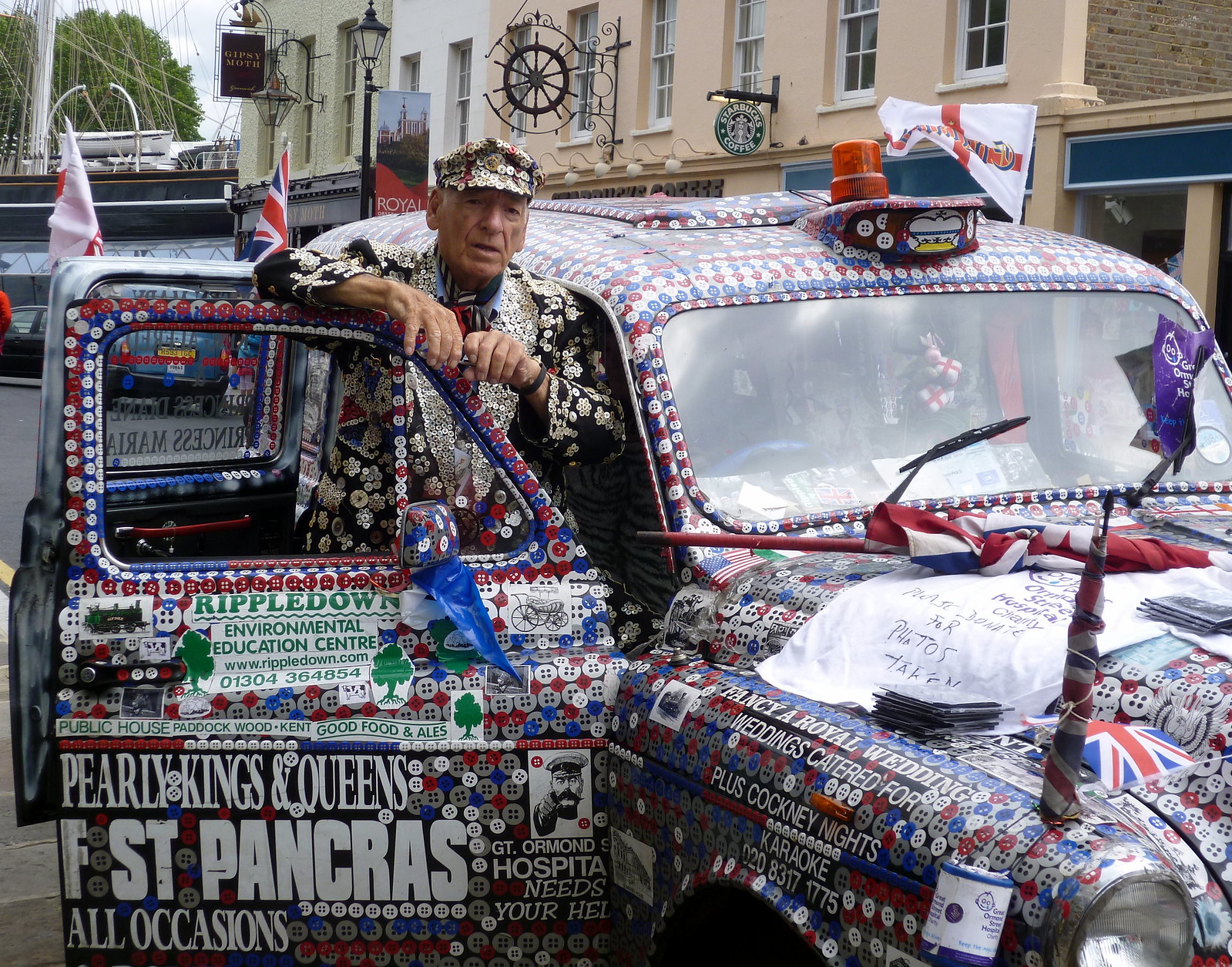This vibrant color photograph, taken in landscape orientation, captures an elderly man—approximately 70 years old—standing beside the open driver's side door of a British taxi that is extravagantly adorned. Both the man and his vehicle are lavishly embellished with red, white, and blue buttons, suggesting a deep admiration for British culture. The man, who is dressed in a black, bedazzled military-style jacket and a matching hat completely covered in buttons, is exiting the taxi which features dense imagery and text related to British heritage. Notable inscriptions include "Pearly Kings and Queens," "St. Pancras," and "Fancy royal weddings catered for," highlighting his apparent enthusiasm for British royalty. Flags adorn the vehicle in various locations: a white flag in the background, a British flag wrapped around the antenna, a blue flag on the windshield wiper, and a folded flag on the car's front. Additionally, a donation bucket or blue cup is attached to the car. The backdrop reveals a street scene with other cars and pub-style buildings featuring vintage lanterns and store signs, adding a historical and community feel to the setting. This photograph is a striking representation of British cultural pride.